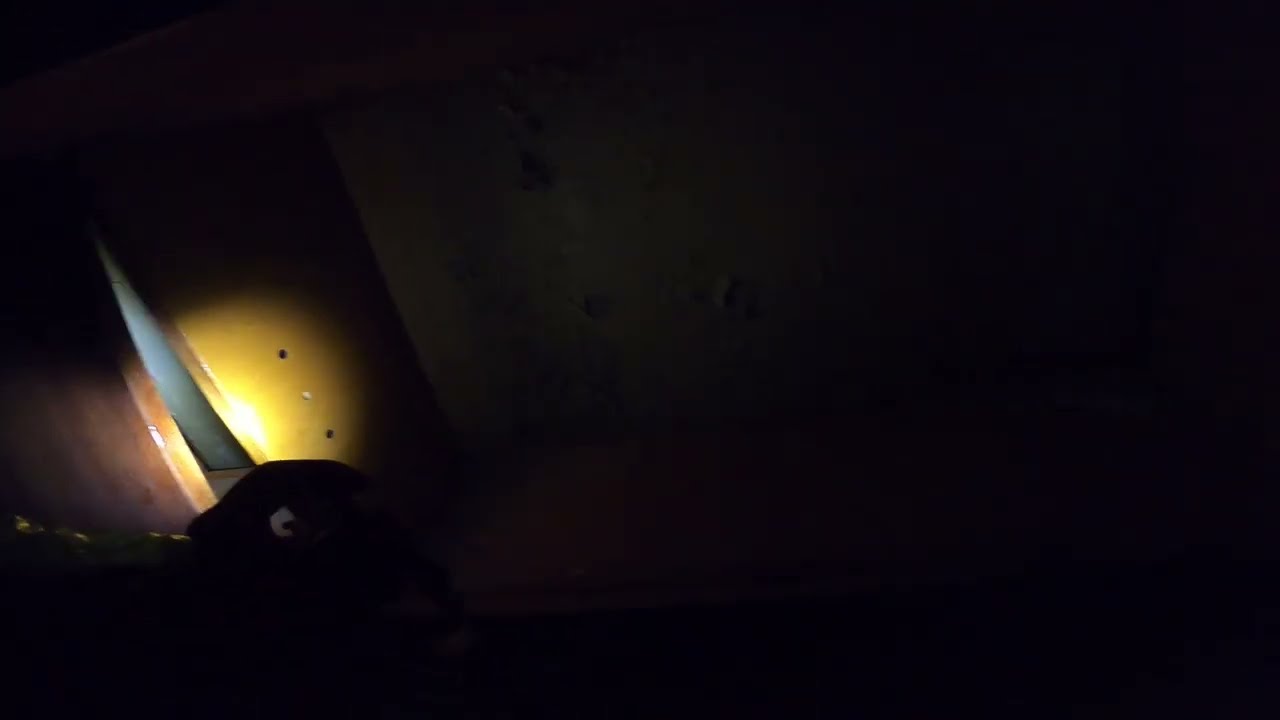The photograph is extremely dark, making it difficult to discern the setting or context. Predominantly black, the image shows a few identifiable features. Towards the left-hand side, there’s a faint light source that emits a golden yellow aura. Underneath this light, there is a round, yellow object with two small black dots, resembling a helmet, with what appears to be a thin silver blade or strap emerging from its bottom. This object is angled diagonally to the left. Nearby, the rough texture of a ceiling or a wooden plank is barely visible, suggesting the photograph might be taken from a crawl space or a dimly lit interior room. To the right, a portion of a cement block comes into view. The ambiguity and minimal lighting leave much of the image open to interpretation, adding to its enigma.